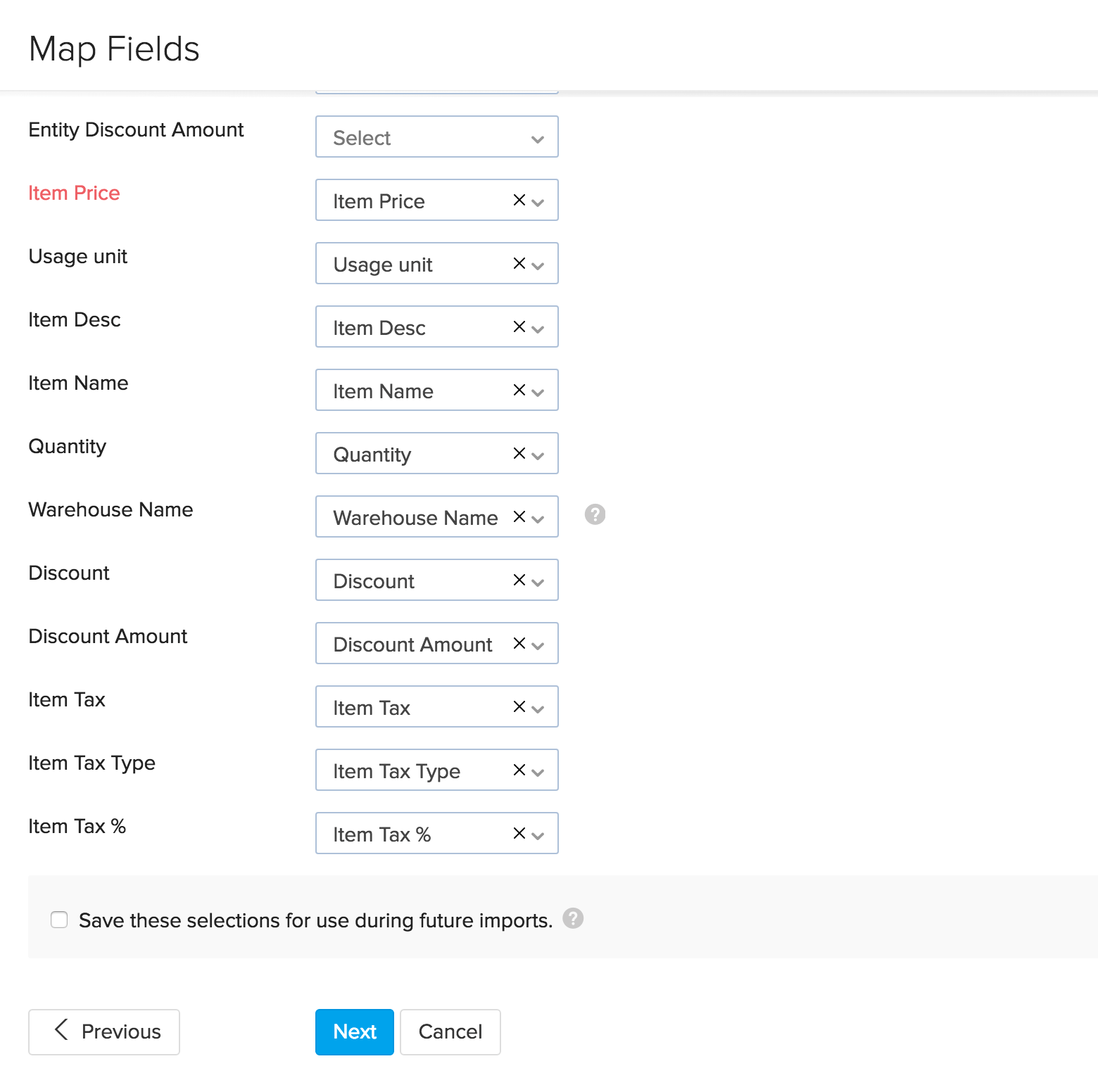The image features a user interface on a white background, titled "Map Fields" positioned on the far left side. There are two adjacent, nameless columns displayed under the title, both uniformly aligned. 

The first column lists a series of field descriptions including:
- Entity
- Discount amount
- Select (highlighted in red)
- Item price
- Usage unit
- Item description
- Item name
- Quantity
- Warehouse name
- Discount
- Discount amount (repeated)
- Item tax
- Item tax type
- Item tax number

The second column contains corresponding drop-down bars for each listed field. The default entries in these dropdowns mirror the field names they correspond to.

At the bottom of these columns, there's a checkbox option labeled, "Save these selections for use during future imports." Directly below the checkbox are three buttons: a "Previous" button, a blue "Next" button, and a "Cancel" button.

The far right side of the image is entirely blank, devoid of any text, images, watermarks, or copyright symbols.